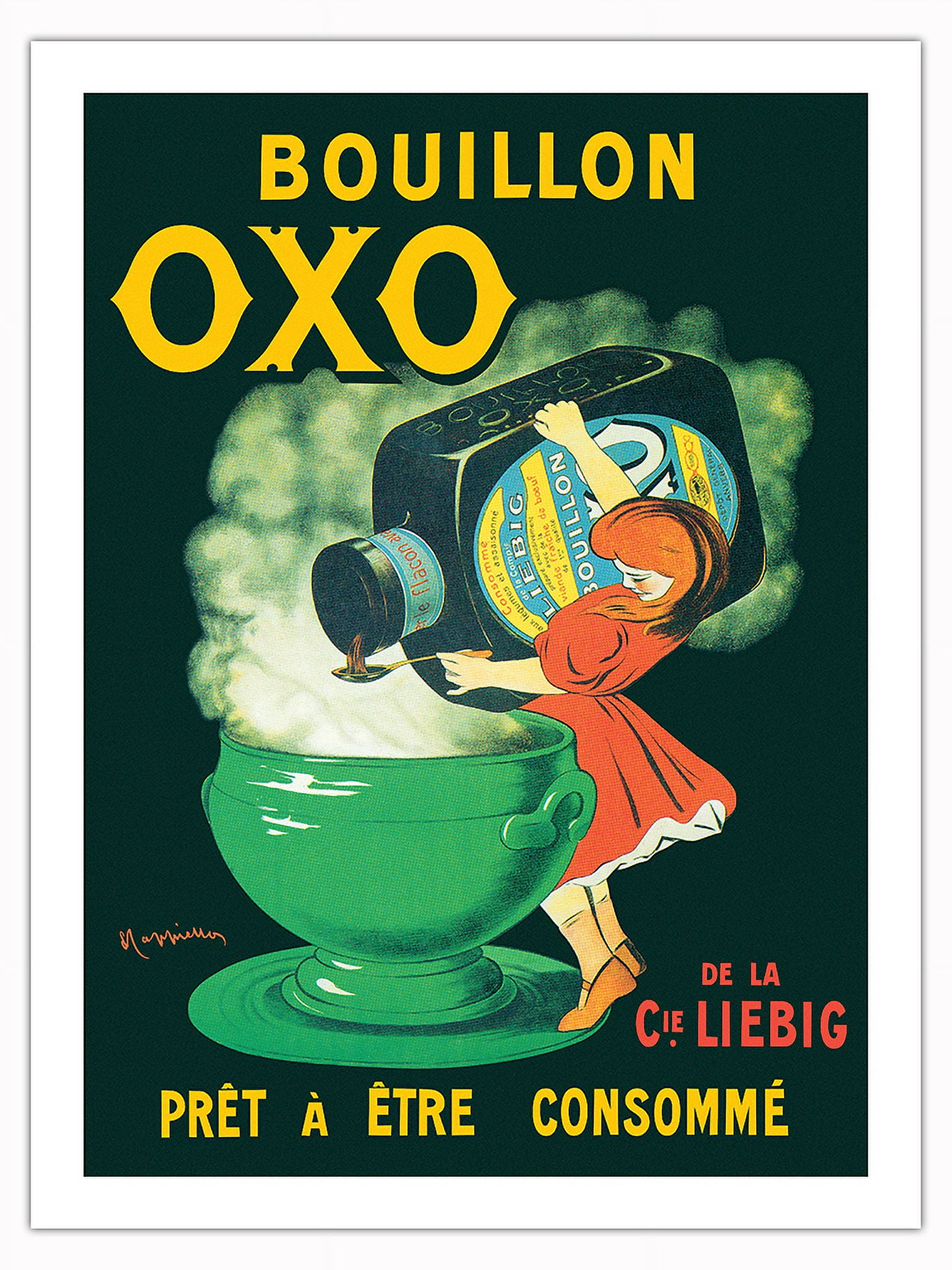This vintage French poster advertises Bouillon OXO. The poster features a deep, dark green—almost black—background, and at the top, in bold yellow text, it reads "Bouillon OXO." The central image is a cartoon-like girl in a red dress with a white ruffle at the bottom and tan shoes, pouring bouillon from a giant, dark bottle with a blue and yellow label into a small spoon above a steaming, green teacup. The bottle appears as large as the girl, emphasizing its importance. The girl has long red hair and is standing with her feet on a plate that supports the teacup. At the bottom of the poster, in yellow text, it states "Prêt à être consumé," which translates to "ready to be consumed." Additionally, in green text to the right of the girl, it says "De La Cie Liebig," indicating the manufacturer. This early-1900s style advertisement captures the nostalgic and functional appeal of the product.